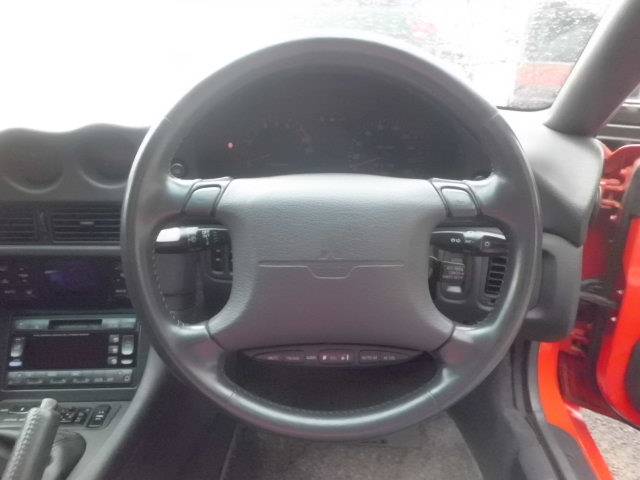The image, taken from the viewpoint of the driver, showcases the interior of a right-hand drive car with a grey, vinyl-like steering wheel prominently featured. The steering wheel, which appears quite old with black knobs on the side controlling the wipers, includes various buttons and two horn buttons, but no logos are clearly visible. The interior of the car is predominantly grey, contrasted by the partially open door, which reveals an orange-red exterior. The centre console is visible, housing a CD player or radio, air conditioning vents, and several functional buttons. The handbrake is positioned on the left side of the image. Due to a combination of bright lighting and dirt on the windshield, the view outside is obscured, though some distant trees can be faintly seen through the glare. The nostalgic, somewhat dated feel of the car's interior suggests it might be from the 1990s.